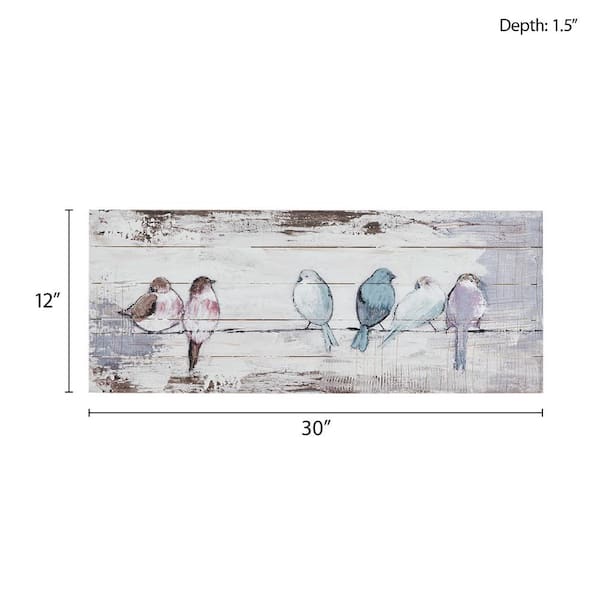The image showcases a detailed, whimsical drawing on a weathered, white-painted wooden panel measuring 30 inches in width, 12 inches in height, and 1.5 inches in depth. The slightly scuffed surface reveals its rustic charm, possibly evoking an old barn wood aesthetic. Sitting on a black line resembling a wire or branch are six different birds, meticulously painted in vibrant colors and varied sizes. The two birds with red tummies and brown accents, likely representing a pair, catch the eye first. They are joined by two turquoise birds adding a pop of serene blue, and two white birds contributing a crisp contrast. Notably, the bird on the far left is quite plump, perhaps suggesting it is the mama bird. The three birds on the right have their backs turned to the viewer, their heads intriguingly twisted to glance back. This charming assemblage not only showcases bird diversity but also the artistry of creating life-like characters on a piece of reclaimed wood.